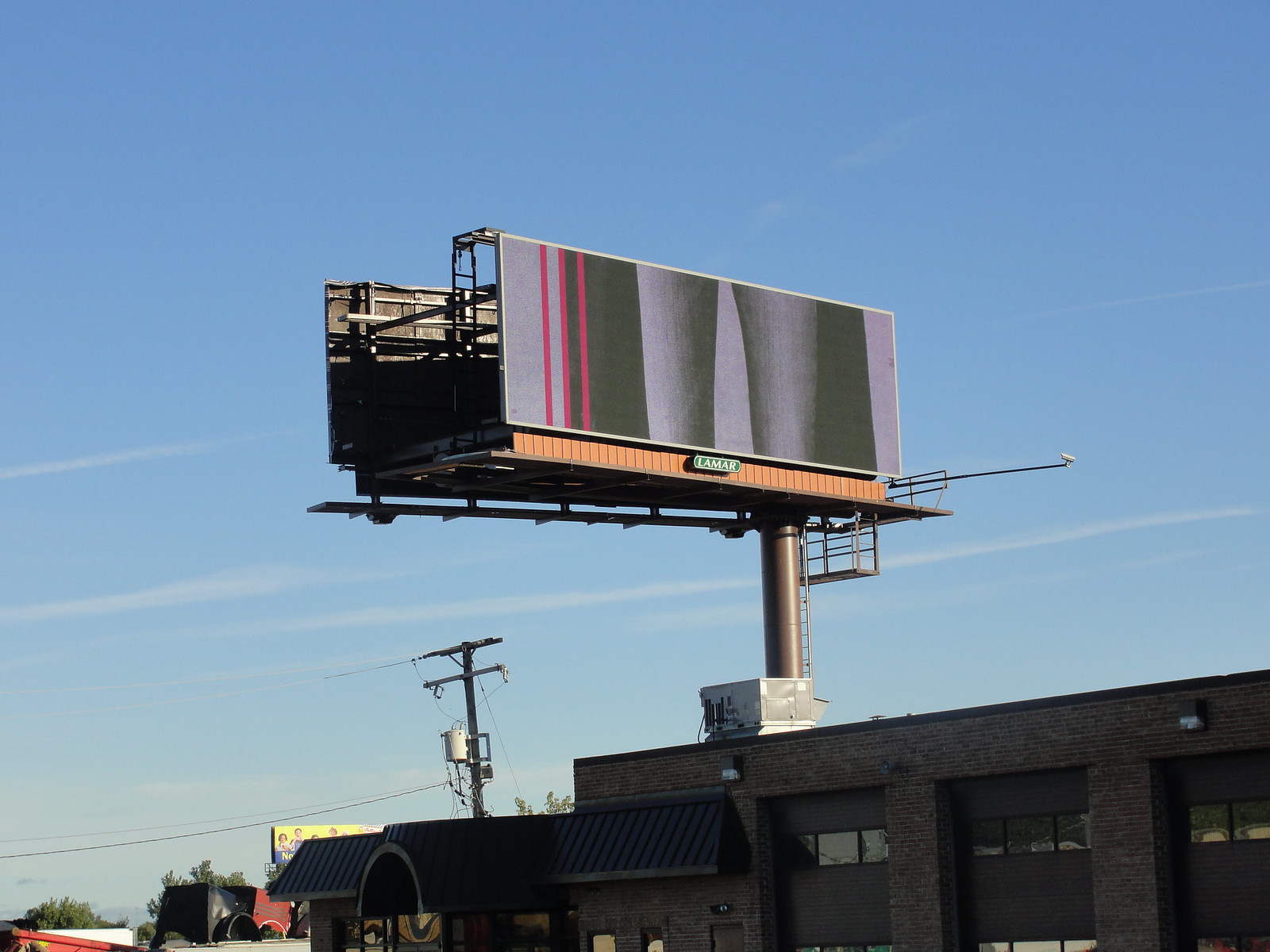The image captures a billboard atop a brown brick building with a blue canopy. The billboard itself features an array of vertical stripes in purple and black hues, with three prominent purple stripes on its left side extending from top to bottom. A large brown pole supports the billboard, accompanied by a ladder and a small platform behind it. Extending from the billboard's right side, another pole with what appears to be a camera at its end is visible. Behind the main billboard, the reverse side of another yellow billboard peeks into view. The building below showcases gray garage doors with three windows each on the top row, and just visible, the tops of three additional windows below the canopy. On the roof of the building, there is a significant air conditioning or HVAC unit. The sky above is bright blue streaked with thin white clouds, and a power line crosses left to right just above the building but below the billboard, adding to the urban atmosphere.